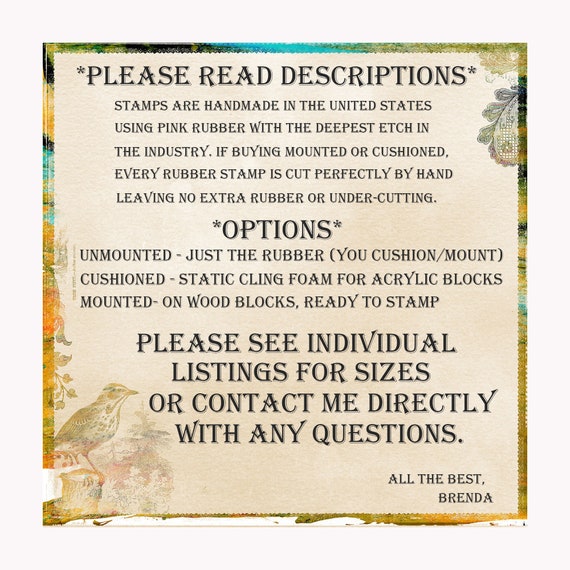This vibrant sign features colorful bordering in shades of yellow, orange, and blue, with intricate green leaves in the top right corner and a detailed illustration of a bird perched on a limb in the lower left. At the top, bold black letters read, "Please read descriptions," followed by smaller text detailing that the stamps are handmade in the United States from pink rubber with the deepest etch in the industry. It promises precision in cutting each rubber stamp, ensuring no extra rubber or undercutting. Below, a section titled "Options" with asterisks on either side lists various purchase choices: unmounted (just the rubber), cushioned (with static cling foam for acrylic blocks), and mounted (on wood blocks, ready for stamping). The sign concludes with a note in bold letters advising viewers to refer to individual listings for sizes or to contact Brenda directly with any questions.